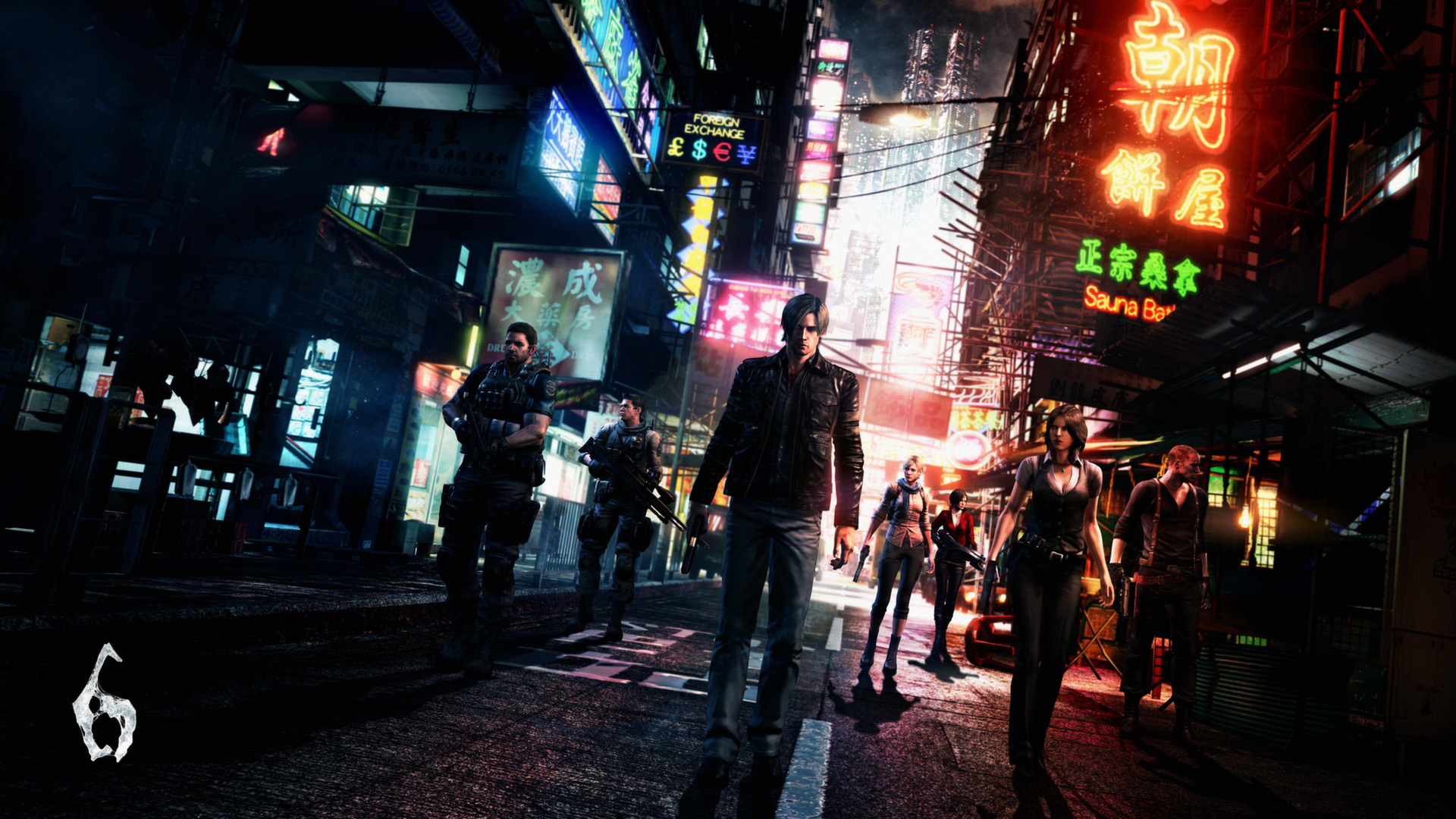The image depicts a dark, neon-lit urban street, presumably set in an Asian city, possibly Tokyo or a fictional metropolis infused with elements from various East Asian cultures. The scene has the distinct, vibrant ambiance of a video game or animated film, dominated by an array of neon signs in vivid colors — oranges, greens, pinks, purples, and blues. Prominent among these signs is one advertising “foreign exchange,” listing currencies like pounds, dollars, euros, and yen. Another notable sign, written in both English and Mandarin, marks a building named “Sauna Bar.”

Despite the colorful neon lights illuminating the buildings, the street itself remains ominously dark. The background showcases tall buildings with their tops shrouded in darkness, while the lower sections glow with a gradient of green, pink, and bright white lights from various neon sources. A closer look at the bottom left corner of the image reveals a small icon, possibly of a goose, and a white marking that resembles the number six.

In the foreground, a group of five individuals exudes an intimidating presence, reminiscent of characters from a high-stakes action movie or crime thriller. The central figure, a man in a leather jacket, stands with a pistol in his right hand, his chin slightly tucked. Flanking him are individuals clad in dark, military-style gear; the ones on his right hold rifles, reinforcing a menacing vibe. On his left, two women similarly dressed in tactical yet somewhat civilian attire, suggest a mix of street and combat readiness. All the figures advance toward the camera with serious expressions, hinting at an imminent, perhaps nefarious, purpose in their stride.